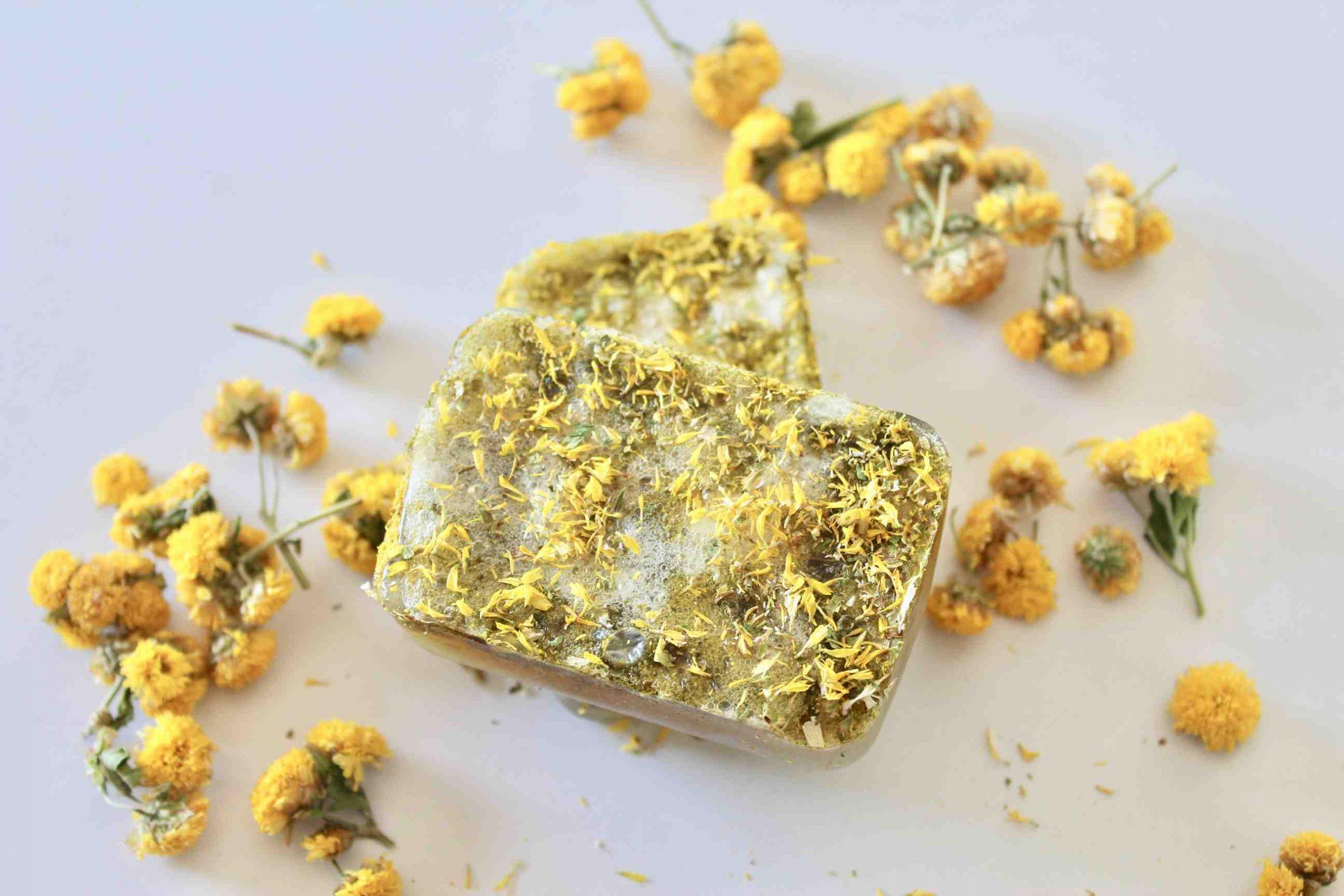In this detailed image, we see two handcrafted bars of soap prominently displayed. The foremost bar is angled slightly from the top left to the bottom right, revealing its intricate design. Both bars feature a rich mixture of beige and gray matter within, and are adorned with crumbled chrysanthemum petals scattered on the top, which impart a textured look. The top bar partially covers a second bar in the background, which is similarly detailed.

Surrounding the soaps are numerous small, yellow chrysanthemum blossoms with green branches and leaves, resembling fluffy pom-poms. These flowers are more densely gathered at the bottom left and upper right corners, while others lie scattered across the white surface on which the soaps rest.

The background is artistically divided diagonally, with a soft pink hue toward the bottom and a light blue hue at the top, enhancing the overall aesthetic. The photograph, rendered in a realistic, food photography style despite the subject being soap, captures the scene in a landscape orientation, providing a top-down view that highlights the organic and artisanal qualities of the soap and chrysanthemums.